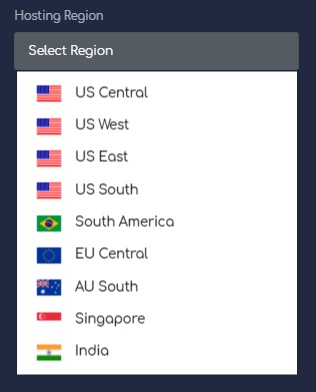The image showcases a selection menu for hosting regions, framed with a black border and titled "Hosting Region" in gray text at the top. Below the title, a gray rectangular box with the text "Select Region" in white serves as an interactive prompt. The menu contains a series of country flags arranged vertically, each associated with a specific region:

1. **United States**: Four flags sequentially representing different regions within the US—US Central, US West, US East, and US South—all depicted with the American flag.
2. **Brazil**: A single flag, resembling Brazil's, labeled "South America."
3. **European Union**: A blue flag adorned with yellow stars arranged in a circle, labeled "EU Central."
4. **Australia**: The Australian flag labeled "AU South."
5. **Singapore**: A red flag featuring a white crescent moon and stars, labeled "Singapore."
6. **India**: The tricolored flag of India, with orange, white, and green horizontal stripes and an indistinct symbol in the center, labeled "India."

The arrangement implies a selection process where a user can choose their respective region for hosting services.